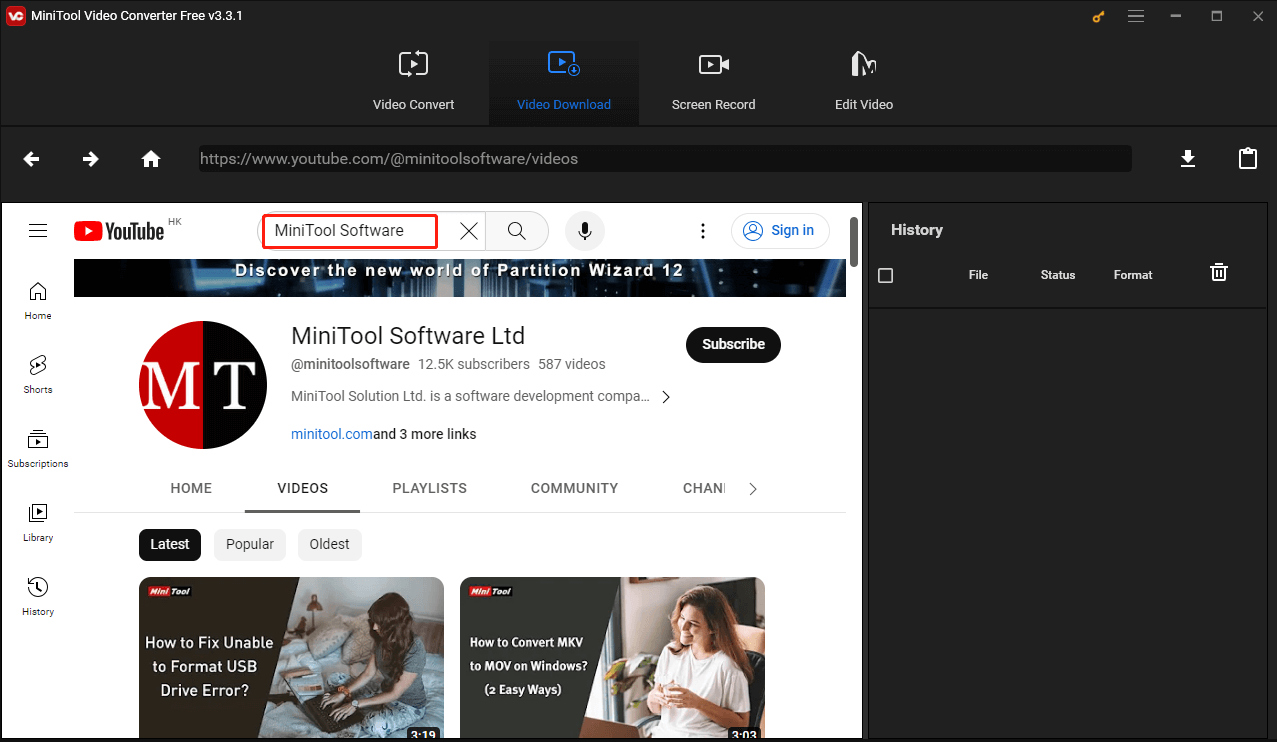The image showcases a section of the MiniTool Software YouTube channel interface. This channel appears to be a valuable resource for content creators, featuring various tools such as a video content box, video download box, screen recorder, and video editing options. The screen is currently focused on the video download feature, highlighting its utility for modifying videos. A small screenshot appears on the webpage, which seems to be associated with their YouTube channel or website design.

The MiniTool Software logo, boxed in red, prominently features the text, "Discover the New World Partition Wizard 12." Alongside the "MT" emblem, the image displays "MiniTool Software LTD" and additional information about their subscriber count and video content.

Further, MiniTool Software LTD is identified as a software development company. The channel's homepage includes videos such as "How to Fix Unable to Format USB Driver Errors" and "How to Convert MKV to MOV on Windows." Additional navigation tabs include Playlist, Community, and Channel, but the user is currently not signed in, so community interactions and channel customizations are not visible.

On the left side of the YouTube interface, the standard navigation options are present: Home, Shorts, Subscriptions, Library, and History, with the latter showing no recent activity. The right side of the screen remains blank, indicating no additional content or suggestions at this time.